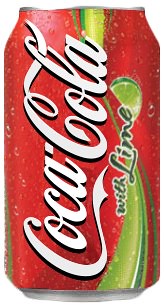This image is a digital illustration of a Coca-Cola can, which appears to have been digitally manipulated or enhanced. The can is predominantly red, featuring the iconic Coca-Cola logo in white, italicized script running vertically up the length of the can, requiring a 90-degree anti-clockwise head tilt to read. Just below the logo, also in a vertical orientation, the words "with lime" are written in a green script font outlined in white. To the right of this text, there is a small illustration of a green lime wedge. 

A wavy, green ribbon-like stripe flows from the bottom of the can upwards, intersecting with streaks of various shades of green and a central white stripe. A notable detail is the undulating, wobbly top edge of the can, suggesting a less-than-perfect digital edit or touch-up. The presence of water droplets covering the surface of the can indicates it's cold and adds a realistic touch. The silver aluminum top and bottom edges are slightly visible on the sides, framing the entire composition and enhancing the overall polished, yet digitally modified, appearance.